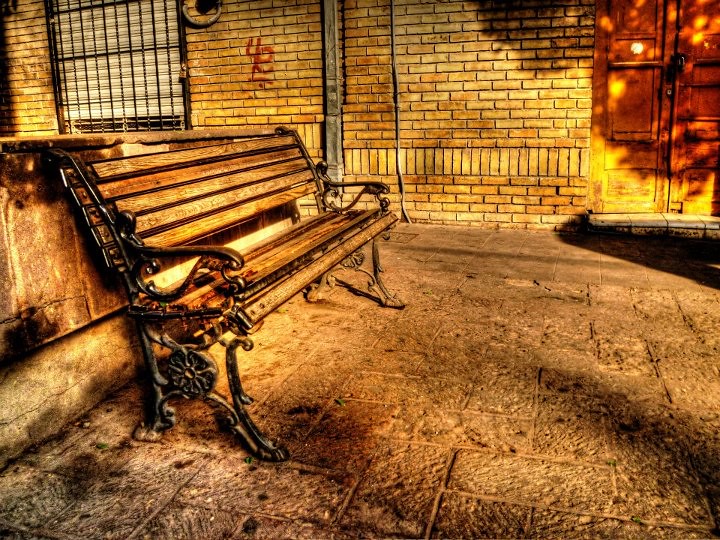The image presents a dimly lit courtyard with a pronounced brownish-orange tint, possibly due to an HDR effect or a lens cover. Dominating the scene is a traditional cast-iron and wood bench, its brown wooden planks complemented by intricately designed black metal armrests and legs. The bench stands on a ground paved with uniform stone blocks, seamlessly extending up to a stone wall behind it. This wall, a grayish-orange color, matches the courtyard's surface and suggests an old, possibly colonial, architecture.

In the foreground, closer to the bench, a shadow, potentially from a nearby tree, adds a dynamic element to the scene, while an adjacent brick wall anchors the background. The brickwork is marked by a horizontal arrangement with a distinctive vertical band, providing texture to the facade. On the left side of this wall, there's a window secured with black bars and framed by what appear to be white interior lines, possibly Venetian blinds. Graffiti in bold red letters and numbers, reading "4E" underlined, is spray-painted between the window and a large brown door to the right. The door contrasts slightly with the orange hues, further enhanced by the fiery yellow light suggesting a setting sun, casting an overall warm glow across the scene.